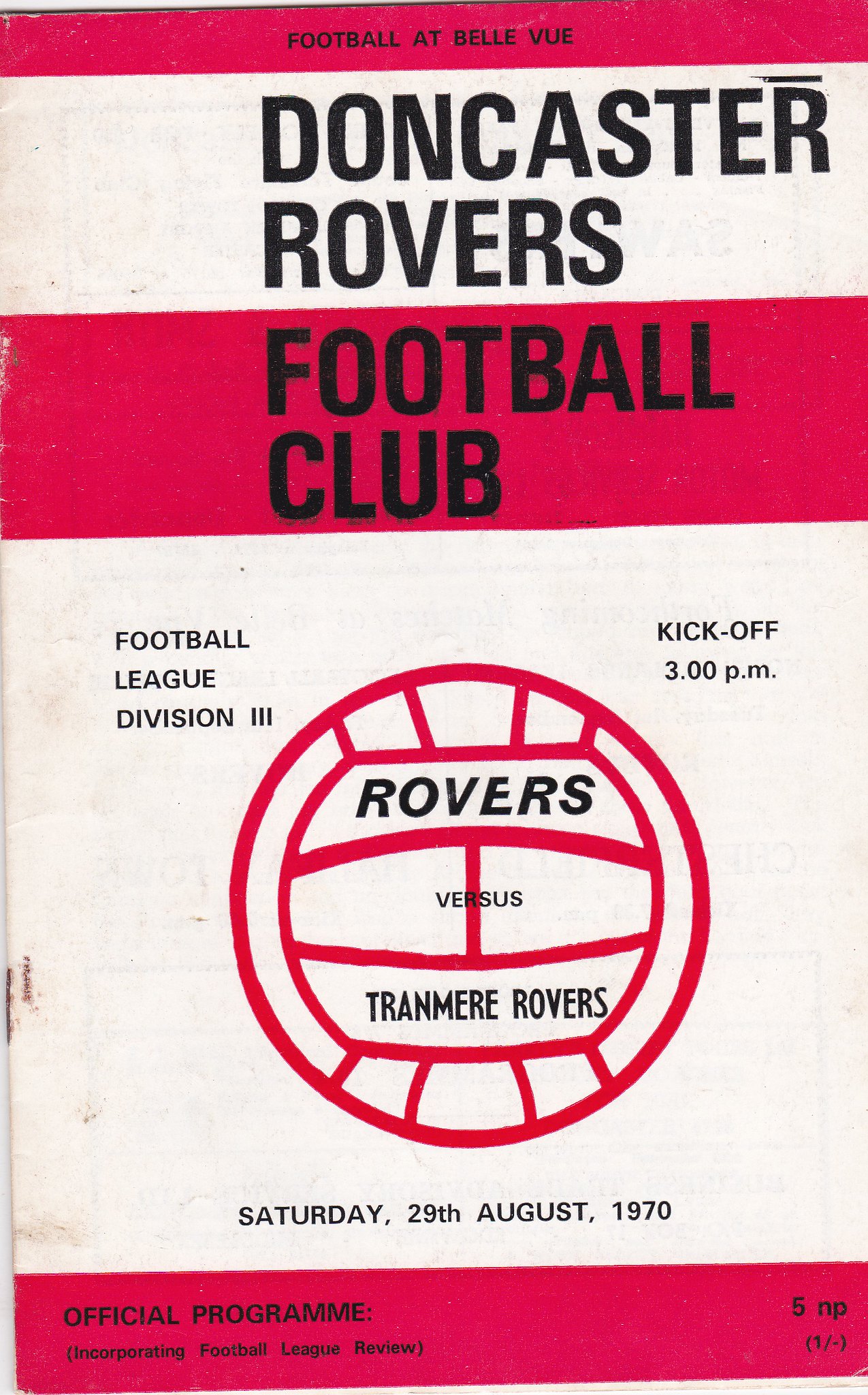**Football at Bally Bowl, Doncaster Rovers Football Club**

This advertisement is for a football match between Doncaster Rovers and Tranmere Rovers, set against a multicolored background dominated by a pinkish-red and beige palette. At the top, "Doncaster Rovers Football Club" is prominently displayed in black letters. Below this, the event specifics are provided: 

In the center, a soccer ball with red lines encircles the details of the match: "Rovers vs. Tranmere Rovers." The game is scheduled to kick off at 3 p.m. on Saturday, 29 August 1970, as part of the Football League Division III. Additional banners provide further information, such as "Football League Division 3" on the top left and "Kick-Off 3pm" on the top right of the soccer ball. The date "Saturday 25 August 1970" is positioned below the ball. Finally, at the bottom of the advertisement, it notes that this is "the official program 5NP," with a mention in brackets incorporating the Football League Review.

The design highlights are consistent and clear, with all text rendered in black, ensuring legibility against the backdrop. The composition is carefully structured to prioritize the details of the event itself.